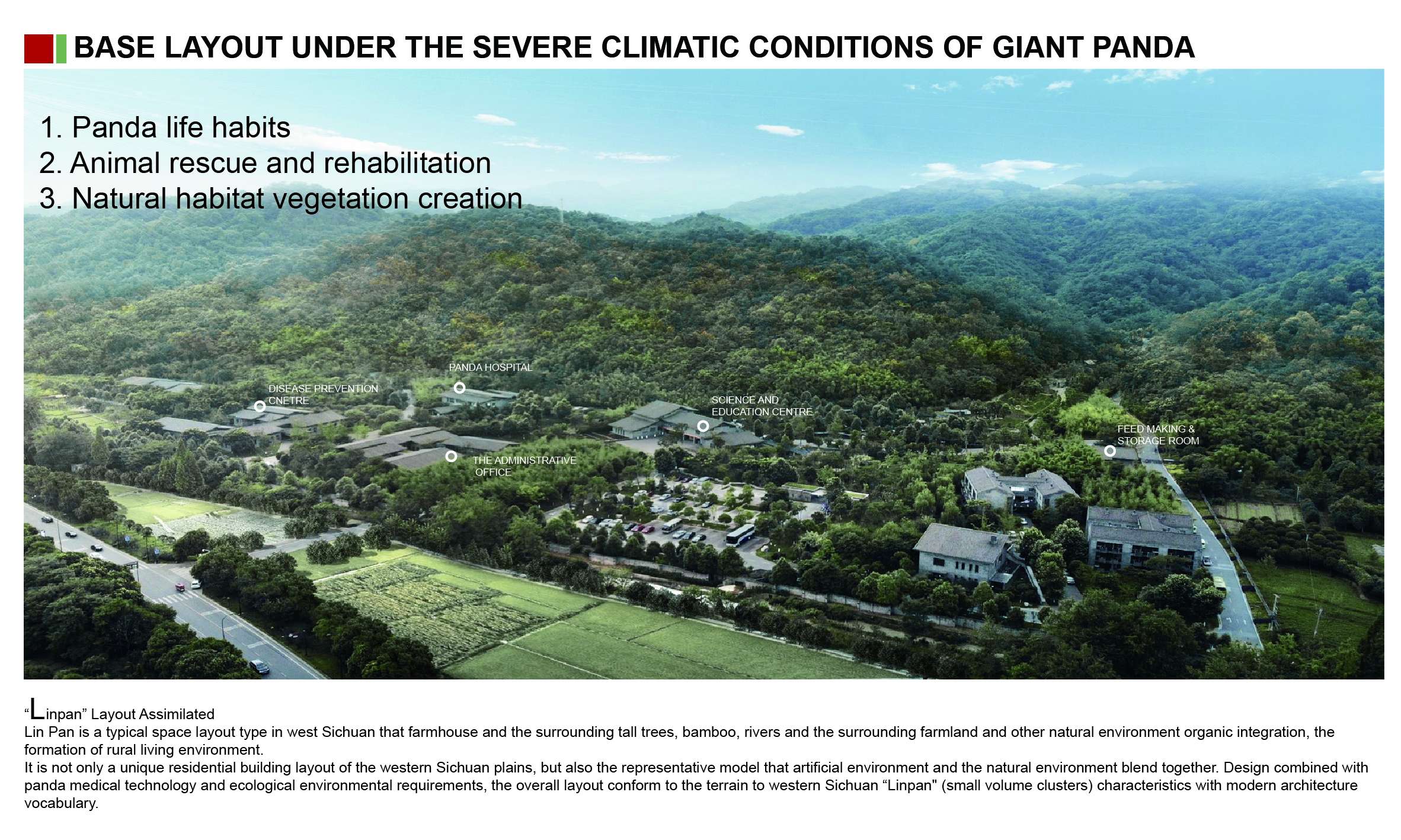This informational poster, titled "Base Layout Under Severe Climatic Conditions of Giant Panda," features a detailed depiction of an area dedicated to panda conservation and related activities. At the top of the poster is a red square with a green rectangle extending downward, which serves as a visual header. Below this, the title is prominently displayed in black text. The poster includes several bulleted points: "1. Panda Life Habitats,” "2. Animal Rescue and Rehabilitation," "3. Natural Habitat Vegetation Creation," "4. Organic Integration," and "5. The Formation of Rural Living Environment."

The main image provides an aerial view of a compound that includes a variety of structures, possibly a dozen buildings identified by specific purposes such as a panda hospital. The layout shows a mix of white houses with gray roofs, green fields, dense forested areas, tall trees, bamboo, and a river with tree-lined banks. Small black letters underneath the image explain that the layout simulates Linnpan, a typical space layout type in West Sichuan known for blending artificial environment with natural surroundings. This design integrates panda medical technology and ecological requirements while reflecting the traditional architectural vocabulary and small cluster formations characteristic of Western Sichuan Plains. The poster emphasizes how the region's unique rural living environment harmonizes with modern needs and the natural terrain.